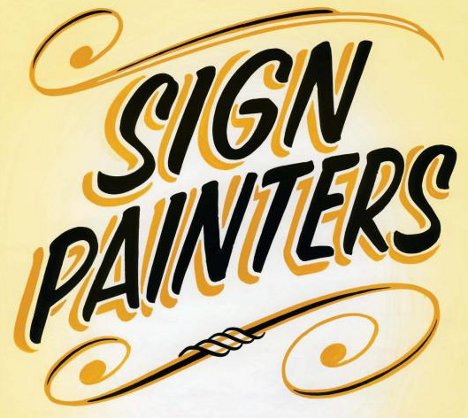The image is an illustration featuring a predominantly yellow theme with a white center. It prominently displays the words "Sign Painters" in informal, bold, black handwritten-style letters. These letters are shadowed by a mustard-colored yellow to create a 3D effect. Above the text is an ornate flourish that swoops over and curves around in a yellow and brown gradient, resembling a partially closed circle that waves across. Below the text, another flourish curves and swirls below the word "Painters," featuring intricate filigree-like decorations with yellow and black accents, including two curly cues with gold balls at the tips and black tendrils in the center. The background surrounding the central white area is a pale gold, complementing the overall graphic design.